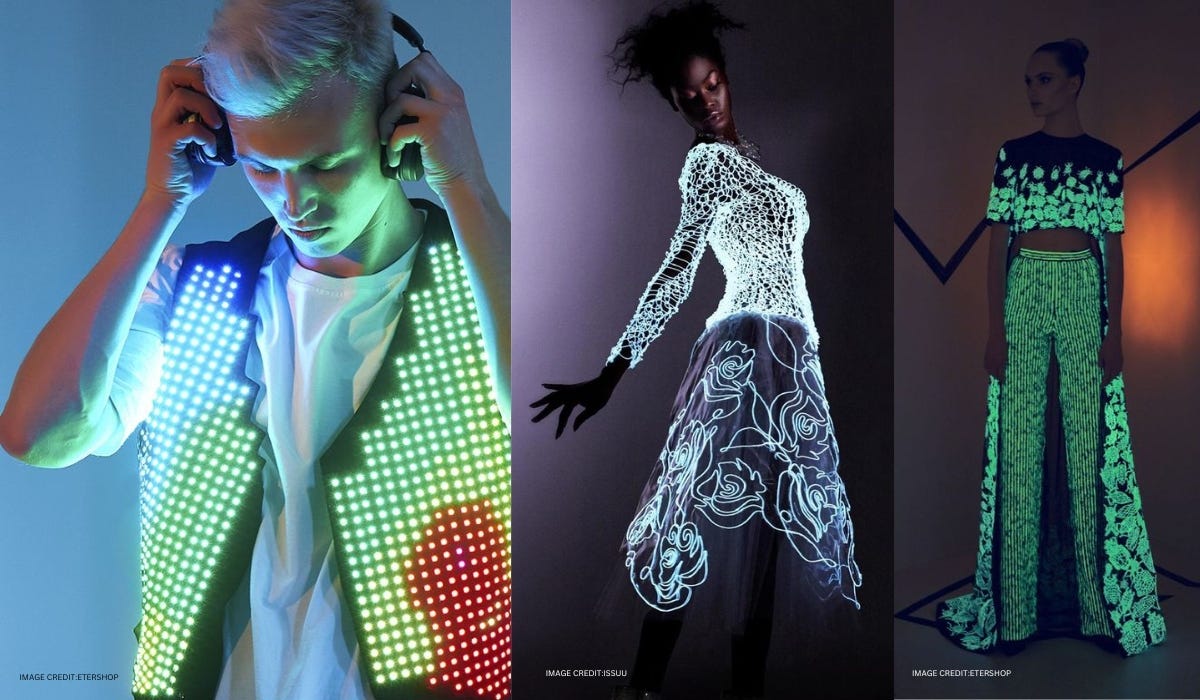The image is composed of three distinct panels, each featuring a unique individual modeling vibrant and contemporary neon outfits, set in varying lighting conditions. In the left panel, a young man with striking blonde hair is seen either putting on or taking off headphones, his hands holding the cups against his ears. He is clad in a white T-shirt topped with a vividly illuminated vest covered in neon green and red square lights, which form a checkerboard pattern lighting up his face.

The middle panel showcases a young black woman with her hair styled up. She is elegantly dressed in a white jersey-like top with extended sleeves that flows seamlessly into a long, black skirt adorned with intricate white patterns, including squiggly lines and floral motifs that reach just below her ankles. Her right hand extends out towards the left side of the frame while her left hand is positioned behind her.

In the right panel stands another woman with brown skin, donning a fashionable ensemble. She wears a short, midriff-exposing black and green neon top that ends at her elbows. This is paired with green neon pants featuring vertical stripes, complemented by a flowing robe-like garment behind her that is patterned with black and white designs. She stands on a brown floor against an orange backdrop, gazing off to her right, completing the trio of distinctive and visually striking portraits.